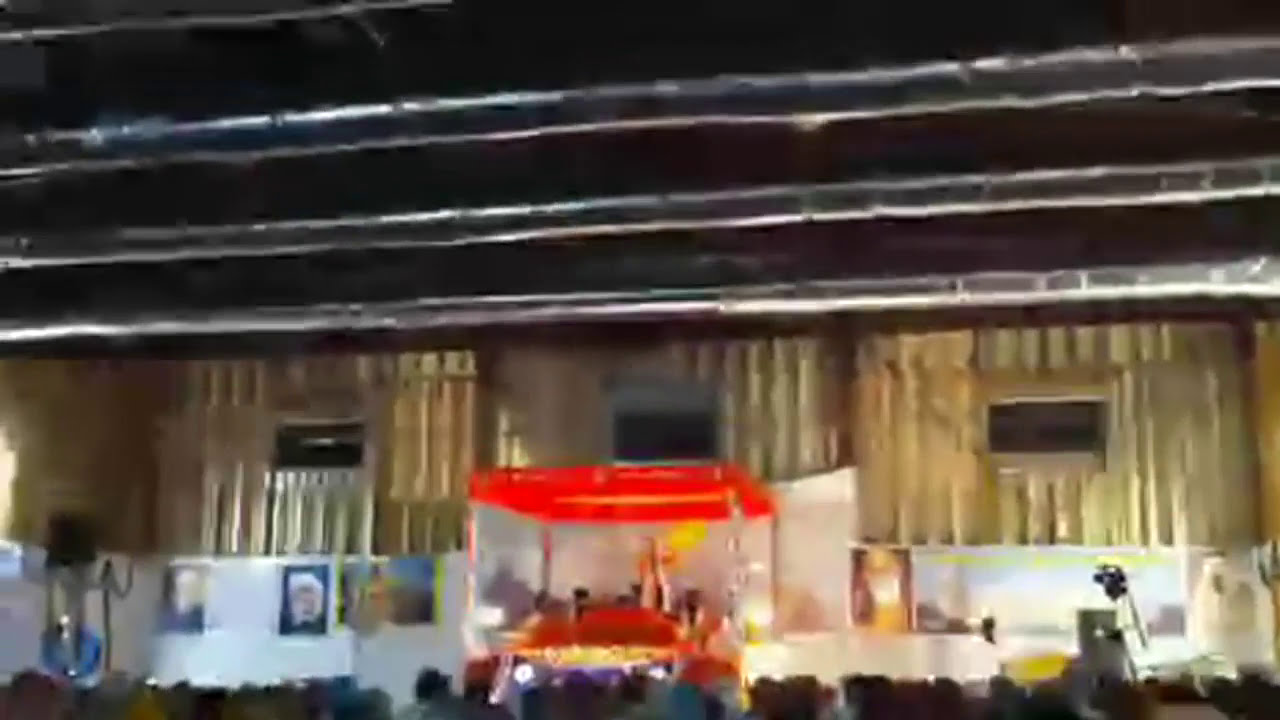The photograph is a low-quality, blurry image of a large event hall taken from the right side of a seated area, pointed towards a stage in the background. The stage, which spans the width of the room, features a central red awning-like structure, underneath which sits a plush red velvet seat. This setup suggests a possible talk or religious ceremony, perhaps by a Hindu spiritual leader, although no individual is currently seated there. The backdrop of the stage includes gold corrugated metal walls divided into three panels, accompanied by three dark windows, likely indicating nighttime outside. The lower portion of the walls is a plain white with several posters attached. Overhead, the ceiling is predominantly black, dotted with exposed pipework and drainage units. In the crowded area, heads of attendees are visible, and there is some technical equipment such as a speaker and camera, indicating the event is being recorded and the speaker’s voice will be amplified for the audience.